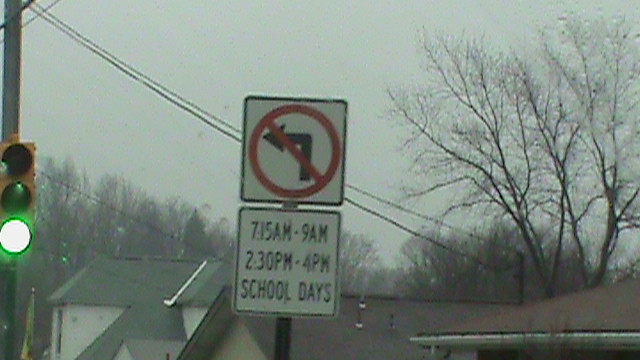In this image, a streetlight is positioned on the left side, with only its green light illuminated, while the yellow and red lights remain off. Above the streetlight, power lines stretch from the top left corner down to the bottom right. The centerpiece of the image is a white square no-left-turn sign marked by a red circle and slash, with a black arrow pointing left. Below this sign, another white square details restricted hours: 7:15 AM to 9 AM and 2:30 PM to 4 PM on school days. The background reveals a dark, cloudy sky, suggesting a dreary, possibly rainy day. Leafless trees and the sloped, paneled rooftops of residential buildings are visible, further indicating it's winter.